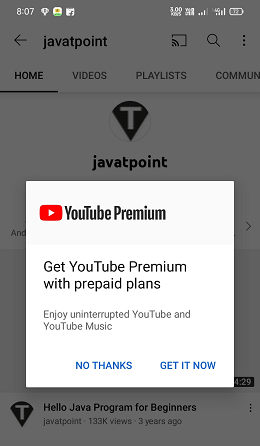This image is a screenshot taken from a person's cell phone, displaying the YouTube app interface. The screenshot captures several distinct elements:

At the top of the screen, the time is displayed as 8:07, and to the right, the battery icon shows a remaining charge of approximately 12%.

The background is grayed out, revealing a partially visible search term entered in the search bar: "JAVATPOINT".

Below the search bar, there is a navigation menu with tabs labeled "Home" (which is currently selected), "Videos", "Playlists", and "Community".

An icon featuring an upside-down triangle with a white "T" in its center is displayed next to the text "Java T-Point".

At the bottom of the screen, there is a video listing titled "Hello, Java Program for Beginners" from the channel "Java T-Point". The video has amassed 133k views and was uploaded three years ago.

A pop-up window is superimposed on the YouTube interface, promoting YouTube Premium. The popup is predominantly white and contains a red square housing a white play icon. The text reads, "Get YouTube Premium with prepaid plans. Enjoy uninterrupted YouTube and YouTube Music." There are two options: "No thanks" and "Get it now".

Notably, the image is in portrait orientation, taller than it is wide, and contains no photographic elements such as people, animals, birds, plants, flowers, trees, automobiles, or bicycles.